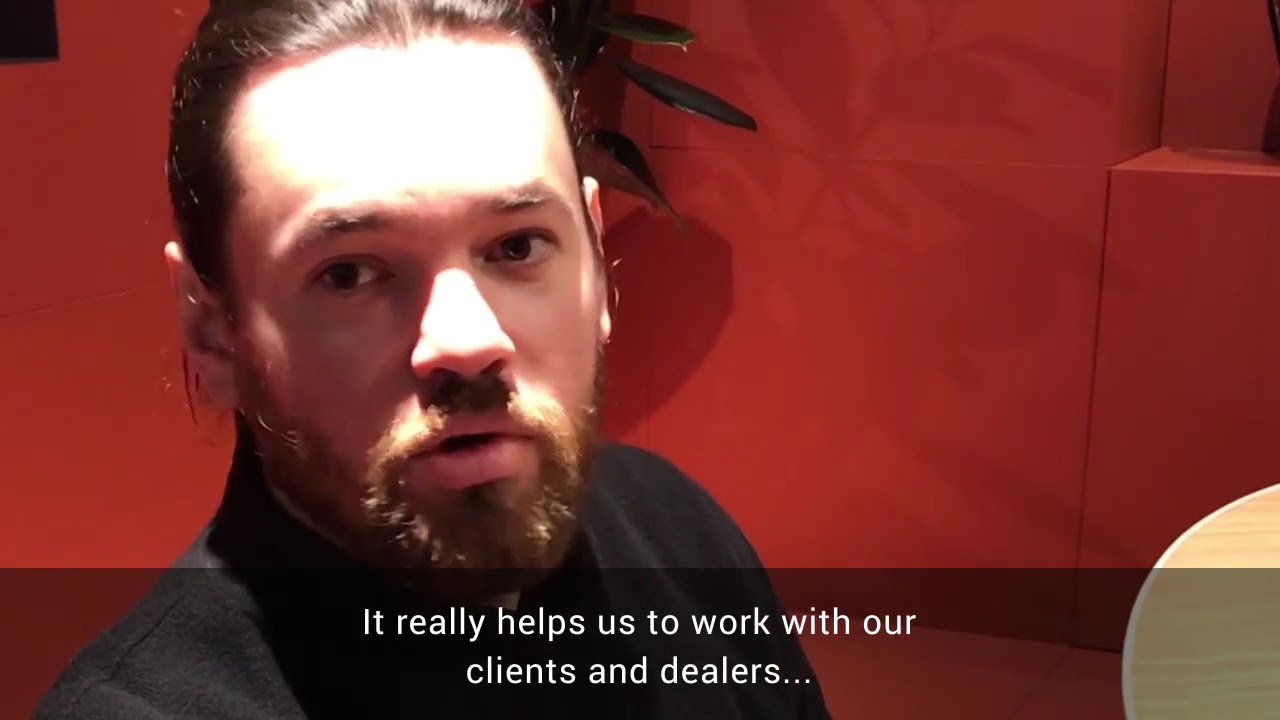The image features a white man standing slightly to the left, wearing a black pullover shirt that covers his neck. He has long brown hair tied in a knot behind his head, a short brown beard, a light brown mustache, and dark brown eyebrows. His brown eyes look directly at the camera. The background is dominated by a vibrant red wall, with a small house plant visible behind his head on the right. A shelf or table is partially seen in the bottom right corner. The floor appears to have tiles, and the overall setting seems to be indoors, possibly for an advertisement or a company website. White text over a transparent black bar at the bottom of the image reads, "It really helps us to work with our clients and dealers." The predominant colors in the image are black, red, white, brown, green, gray, and tan.